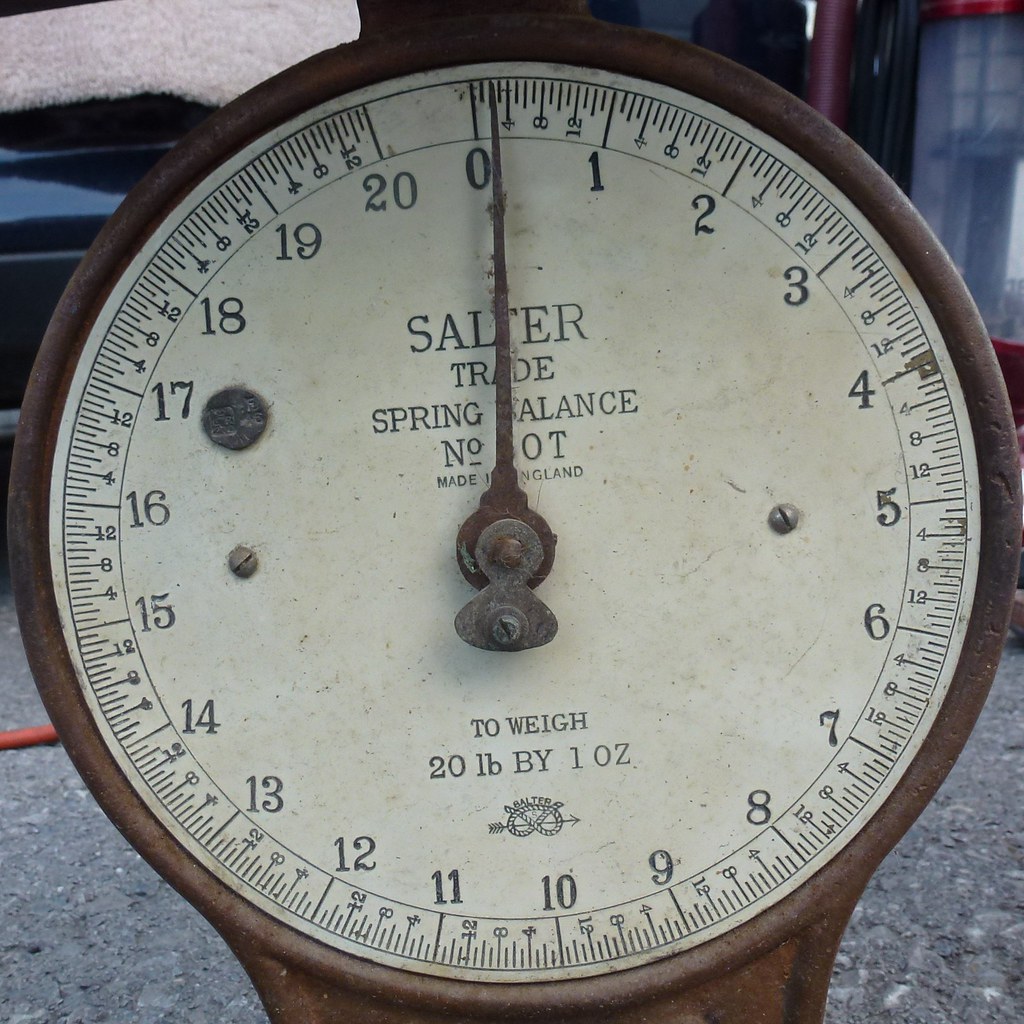This image is a detailed close-up photograph of an old vintage scale, featuring an analog gauge that closely resembles a circular clock. The scale dial starts from zero at the top and goes clockwise, marked by hash marks and numbered increments, reaching up to 20 pounds, with the number 10 positioned at the bottom center. The dial is adorned with black text on a white plate, reading "Salter Trade Spring Balance, Made in England, to weigh 20 pounds by 1 ounce." A prominent bronze-colored needle points to zero, indicating the scale is currently at rest. A distinctive pretzel-shaped logo, labeled "Salter," is also visible on the dial. The scale is set against a backdrop of textured fabric, highlighting its vintage charm and intricate engineering.